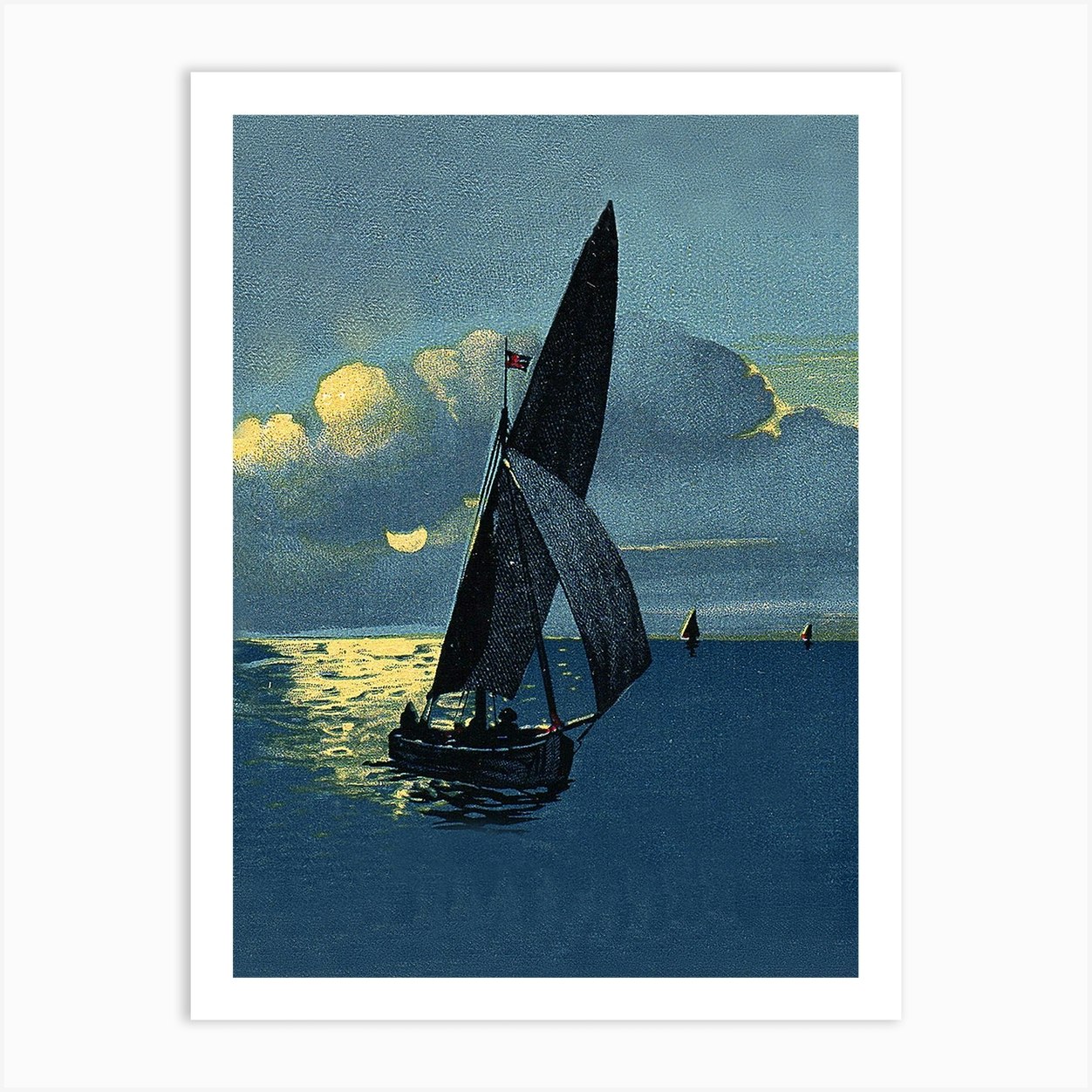This rectangular artwork, prominently hung against a white wall with a thin white border, portrays a moody and atmospheric maritime scene. Dominating the composition is a small sailboat with two billowing sails—indicative of heavy winds—sailing toward the viewer through the dark, inky blue waters, which are sporadically highlighted by a faint glow from a barely visible celestial body. The sky is cloaked in full, billowing clouds, adding to the scene's ominous ambiance. While most observers speculate whether the source of light is the sun or moon, the low light and overall tone suggest it could be a moonlit setting. Additionally, the sailboat carries a blue flag tinged with red, though its precise design remains indistinct. In the foreground, some rocks break the water's surface on the right, indicating shallow waters, while in the background, two smaller sailboats appear on the horizon, adding depth to the scene. There are two or three shadowy figures aboard the main boat, which resembles a working fishing vessel with a mainsail and a spritz sail, moving through turbulent seas under the dim, cascading light from above.